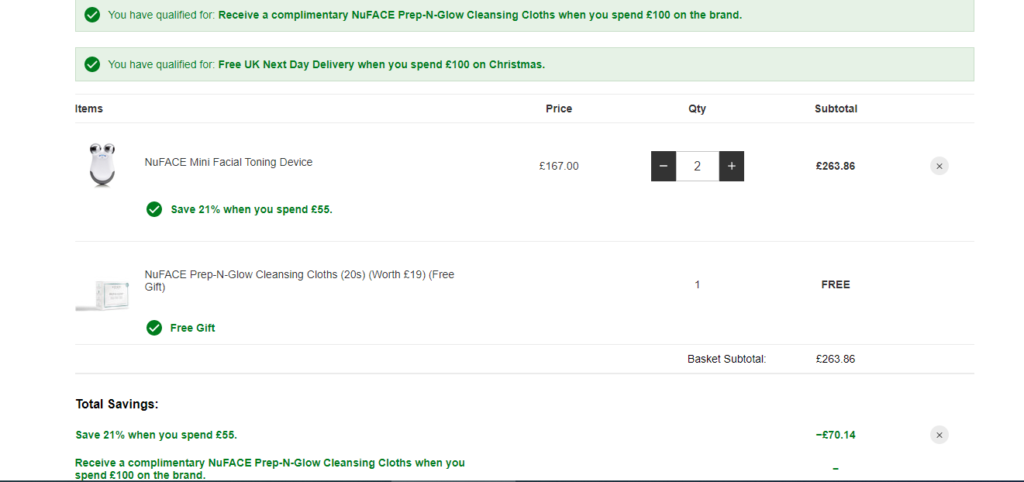**Detailed Checkout Page Screenshot Description:**

The screenshot captures a checkout counter webpage with a detailed overview of the cart contents and summary. At the top, a green box spans the width of the screen, featuring a green circle with a white checkmark on the left, accompanied by some text. Directly below it, another green box similarly stretches across the screen, also containing a green circle with a checkmark and text below it.

Proceeding downwards, the cart's contents are displayed. The header of the cart section lists columns for items, price, quantity, and subtotal. Two items are shown in the cart:

1. **NuFace Mini Facial Toning Device:**
   - **Image:** An image of the NuFace Mini Facial Toning Device is displayed.
   - **Description:** Next to the image, the text reads "NuFace Mini Facial Toning Device."
   - **Details:** Below the description, green text is visible next to a blue circle with a checkmark.
   - **Price:** The price is listed to the right of the details.
   - **Quantity:** A quantity selector box follows, containing black, white, and red boxes. The left black box has a minus sign, the right red box features a plus sign, with the number "2" displayed in the white box in the middle.
   - **Total:** The total cost for this item is shown next to the quantity selector.

2. **NuFace Prep and Glow Cleansing Cloths:**
   - **Label:** A label indicates this as "NuFace Prep and Glow Cleansing Cloths."
   - **Details:** Below the item name, a green circle with a checkmark and the text "Free Gift" is shown.
   - **Quantity and Price:** It is noted as quantity one and free of charge.

Beneath the items, the **basket subtotal** is highlighted according to the quantity, alongside the subtotal amount on the right. Below it, the **total savings** section is displayed, featuring green text on the left describing the savings and a corresponding amount on the right, adjacent to a grey circle with an X in it.